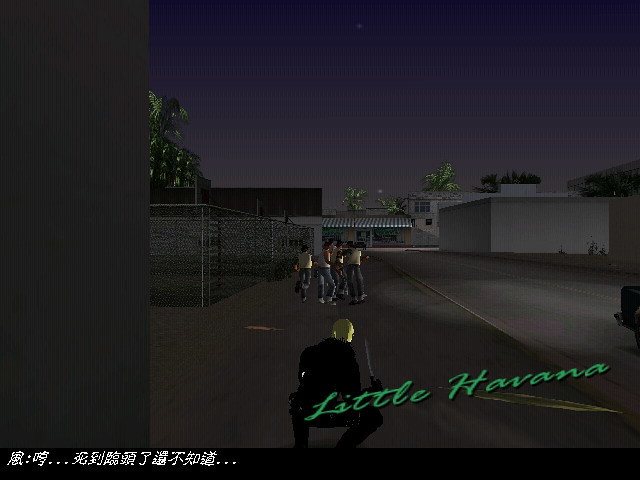In this rectangular image, a nighttime scene reminiscent of a vintage video game unravels with an air of suspense. Central to the composition, a group of five individuals stands circled, each donning denim pants and white tank tops, their postures suggesting a serious gathering. Dominating the foreground, we see the back of what appears to be a central character dressed in black, with a bald yellow head or possibly a helmet or hat. Above this figure's head, in cursive green lettering, the words "Little Havana" are prominently displayed. 

The setting is a darkened street, illuminated sporadically, enhancing the gritty atmosphere typical of urban landscapes. To the lower left, incomprehensible Asian script adds a mysterious element to the scene. On the left side of the image, a chain-link fence runs parallel to the group, while on the right, low-lying white buildings form a stark contrast against the darkness. The tops of silhouetted palm trees peek out from the background, anchored by a pitch-black sky. This visual narrative captures a moment brimming with tension, set against a backdrop that is both enigmatic and evocative.